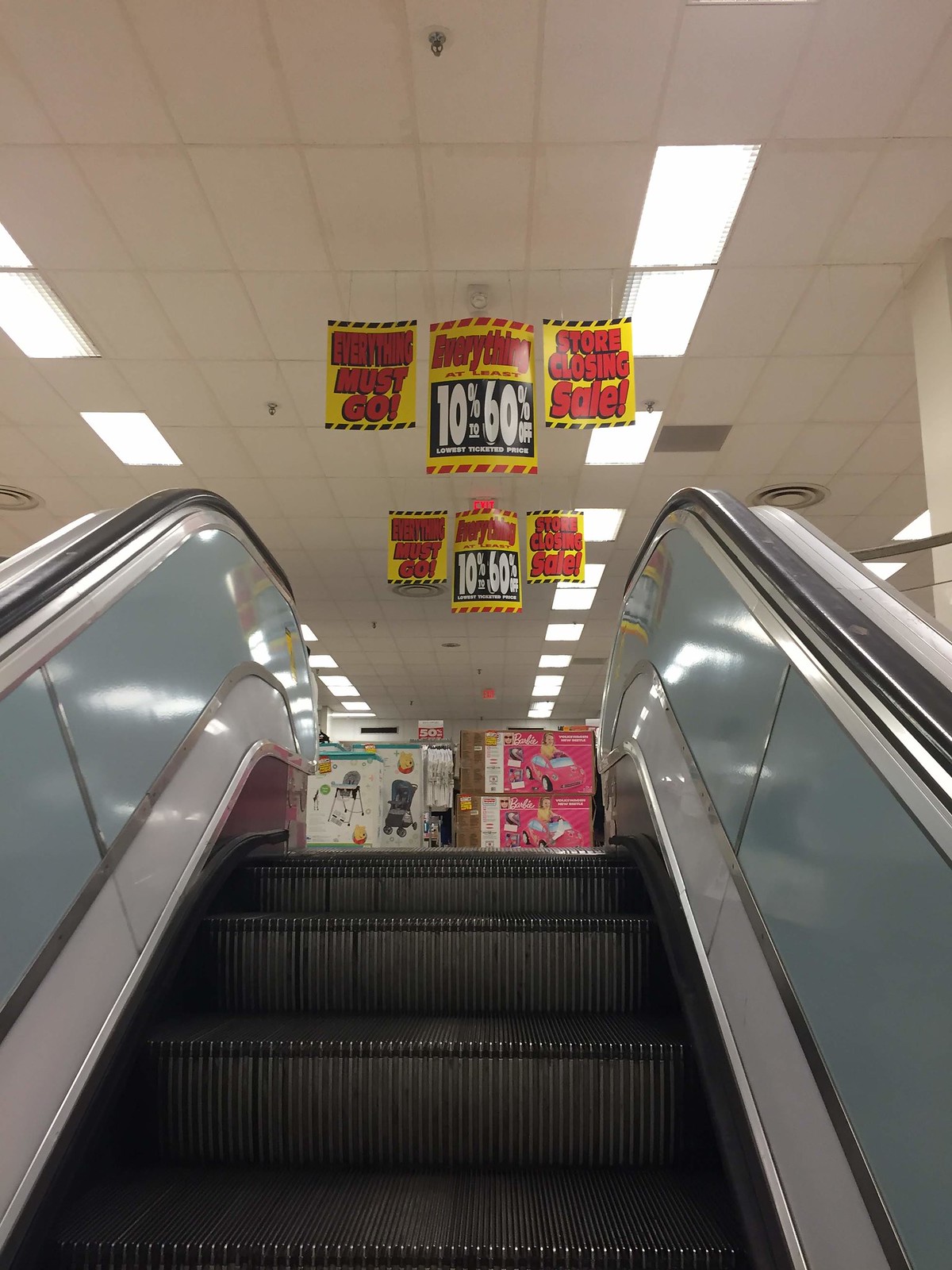The image depicts an escalator with a person ascending it. Overhead, several yellow paper signs are suspended from the ceiling, prominently featuring bold purple letters. One sign reads "Store Closing Sale" with a mixed color palette: the words are predominantly in red while the percentage discounts, "10% to 60% off," are in white. Another sign declares "Everything Must Go," entirely in red lettering. As the viewer's gaze ascends along the escalator, the sides of the escalator rails are visible. At the top, the store floor is cluttered with packages and boxes, creating an immediate obstacle upon reaching the upper level.